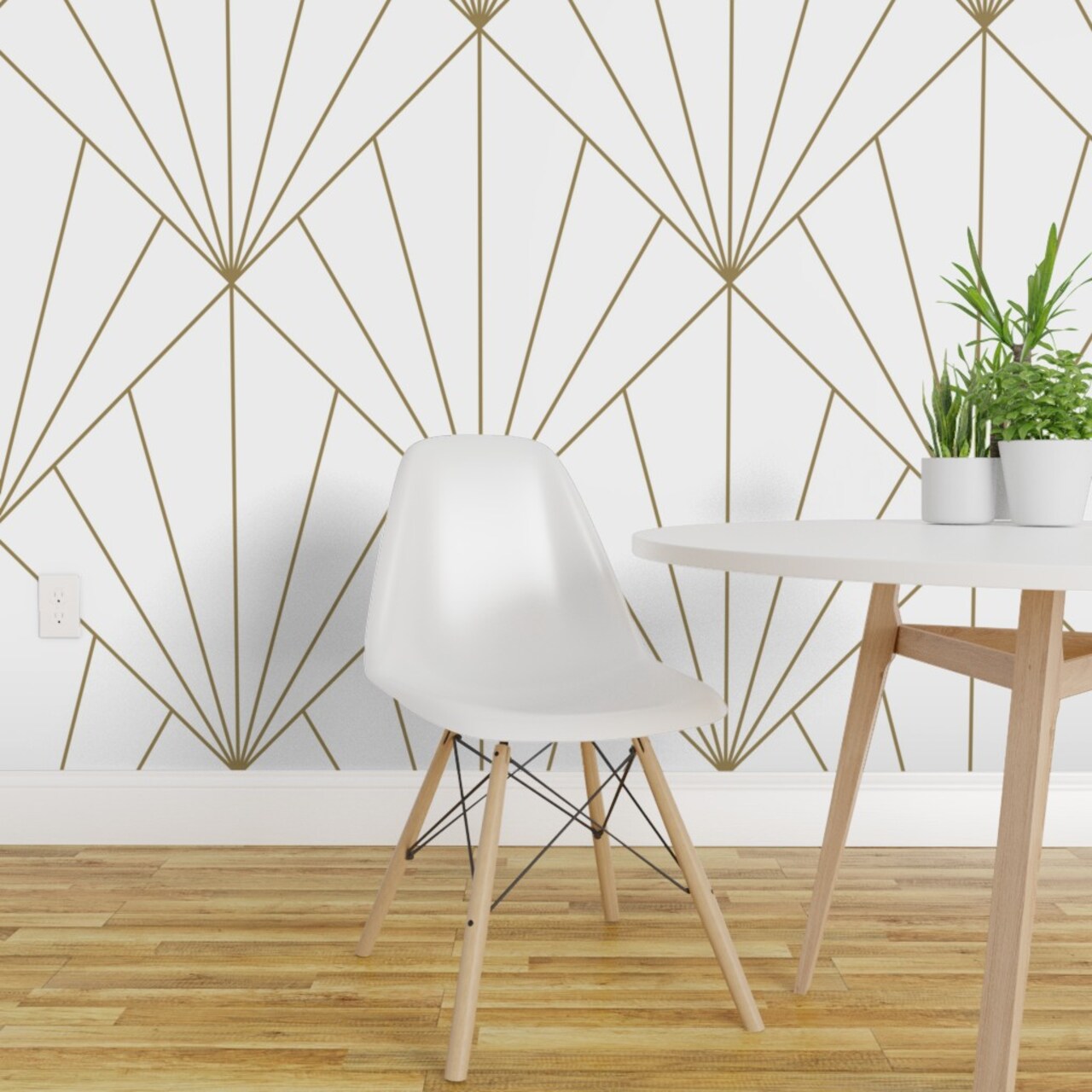The image depicts an interior setting, possibly a living space or an office. Dominating the scene is a white wall adorned with angular, geometric patterns in gold and brown that create a complex and striking visual effect. 

In the foreground stands a pristine white chair, which features grid lines in black, likely for structural support. The top of the chair appears to be made of plastic, while the legs are light beige, wooden or tan-colored metal, connected by black wires to enhance stability. 

Adjacent to the chair, there is a white table with light beige legs that match the chair. Atop the table sit white planters containing vibrant green plants, adding a touch of nature to the setting. 

The flooring is made of rich brown hardwood, grounding the scene with warmth and texture. Tucked subtly within the image, there's an electrical outlet on the left-hand side of the wall, blended into the elegant yet functional decor.